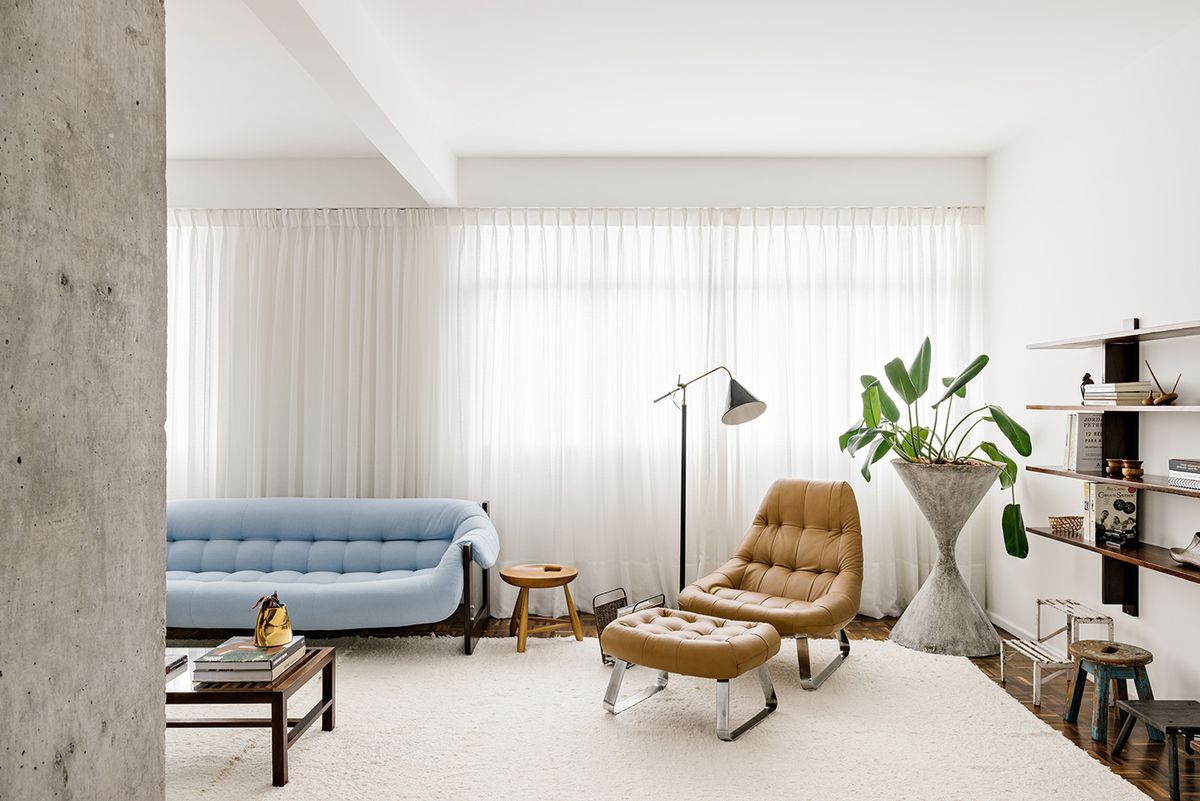This color photo captures a modern living room characterized by its predominantly white decor. The white ceiling and sheer, breezy curtains contribute to the airy atmosphere. Covering most of the parquet floor is a large, white area rug. Dominating the left side of the room is a light blue, plush, rounded sofa with a dark wood frame, positioned near a tan lounge chair and matching ottoman with a silver metal base. To the left of the sofa, a dark brown coffee table holds a book and a house plant. Adjacent to the sofa, a wooden table with a round top and a black remote control adds to the setting. In the left corner, an hourglass-shaped planter with a marble-patterned finish houses a plant with long, green leaves. The right wall features a mounted shelving unit with a black base, wooden shelves, books, and a small brass pot, complimented by a white step ladder and a small round brown table beneath it. The back wall is adorned with a vast window, covered by light, lacy curtains, allowing ample daylight to flood the space. A floor lamp with a green pole and gold accents stands beside the lounge chair. The room's cohesive design is accentuated by thoughtful details and a harmonious color palette.